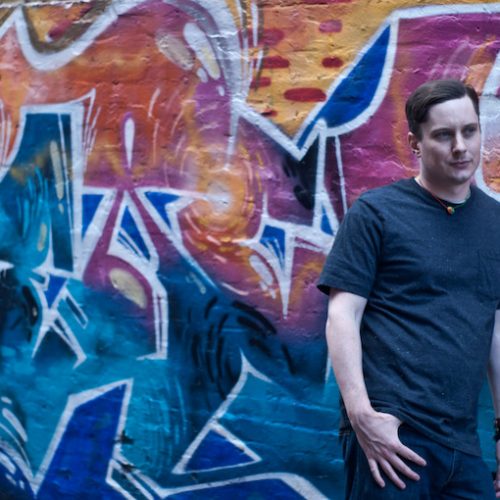In this vibrant square photograph, a man with short, brownish-dark hair, dressed in a short-sleeve dark shirt—either black or dark blue—and blue jeans, stands in front of an expansive, graffiti-covered brick wall. His right arm is slightly out of frame, with his thumb tucked into his pocket and his four fingers resting visibly against his leg. The man is wearing a short necklace and appears contemplative as he looks off into the distance rather than directly at the camera. The graffiti mural behind him is replete with a spectrum of colors—varying shades of blue, white, red, yellow, orange, purple, and black—creating a cohesive and dynamic composition without any empty spaces. Central to the mural is a striking design, featuring a sun-like circle with a spiral around it, evoking the imagery of a galaxy. The top half of the wall features lighter colors, transitioning to darker hues at the bottom. Scattered throughout the artwork are abstract shapes and possibly text, rendered almost unreadable but outlined in a mix of sunset colors and outlined with white. The overall effect is an explosion of color and form, presenting a powerful backdrop to the man's relaxed yet enigmatic presence.